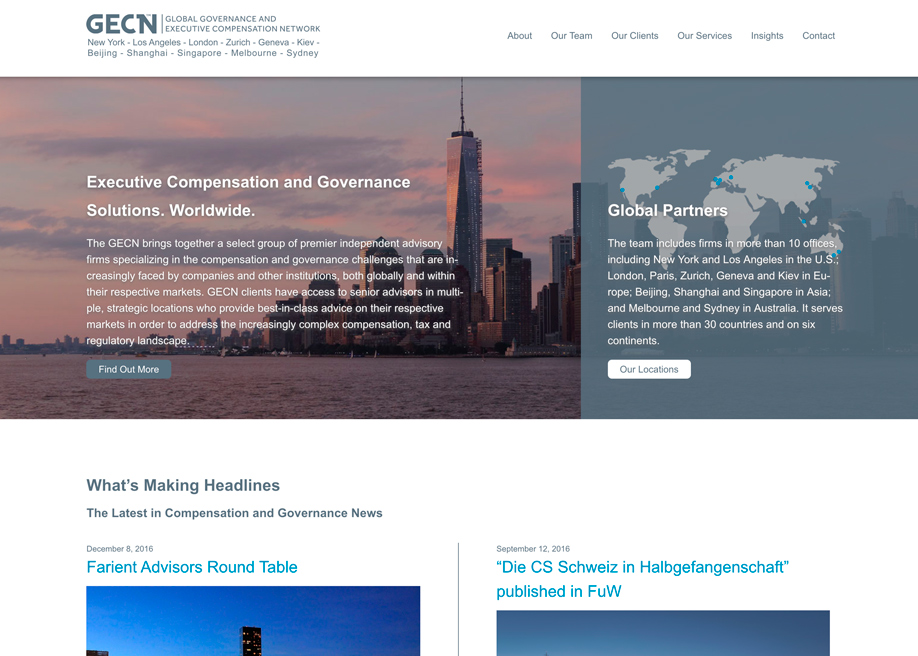The image showcases a comprehensive banner with text and visuals that prominently display the Global Governance and Executive Compensation Network (GECN) branding. 

At the top of the page, set against a clean white background, the text "GECN" is positioned in the upper left-hand corner, followed by the full name "Global Governance and Executive Compensation Network." The header also lists major cities where GECN operates, including New York, Los Angeles, London, Zurich, Geneva, Kiev, Beijing, Shanghai, Singapore, Melbourne, and Sydney. On the right side, navigation options for "About," "Our Team," "Our Clients," "Our Services," "Insights," and "Contact" are visible.

The central image features a serene body of water under a twilight sky decorated in hues of blue and pink. A sprawling city skyline with towering skyscrapers forms the backdrop. Overlaid text reads, "Executive Compensation and Governance Solutions Worldwide."

The description continues, explaining that GECN unites a select group of premier independent advisory firms specializing in addressing global and local compensation and governance challenges. This network provides clients access to senior advisors in strategic locations worldwide, who offer best-in-class advice on complex compensation, tax, and regulatory matters. A call-to-action button labeled "Find Out More" is prominently displayed.

On the right, additional text titled "Global Partners" reveals that GECN comprises firms located in over ten offices across key cities in the U.S., Europe, Asia, and Australia, serving clients in more than 30 countries on six continents.

Finally, a section titled "What's Making Headlines" offers the latest updates in compensation and governance news, featuring topics such as Variant Advisors Roundtables and "DICS Swiss in Fallenfegenschaft," as published in the FUW.